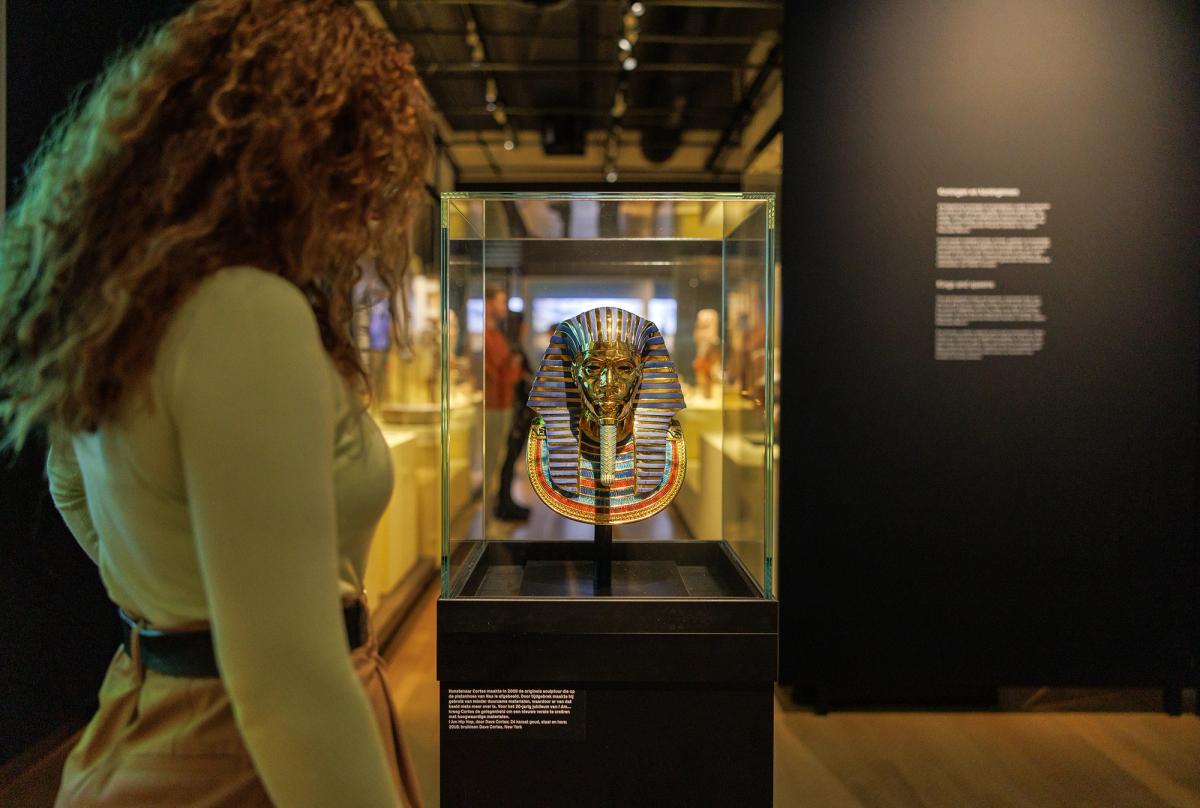The image depicts a woman with long curly hair cascading down her left side, wearing a long-sleeved shirt and leather pants with a belt around her waist. She stands in a museum, staring intently at a glass case that houses a bust of King Tut adorned with a blue and gold headdress and intricate chest decorations, highlighted under museum lighting. The exhibition, titled "Black Culture in Egypt," showcased in the Netherlands, portrays King Tut with an emphasis on Black heritage, and the display has a descriptive pedestal with white text. The museum's walls are black with white text paragraphs illuminated by spotlights. In the background, hardwood floors span out with visitors examining various ancient artifacts in other glass cases.